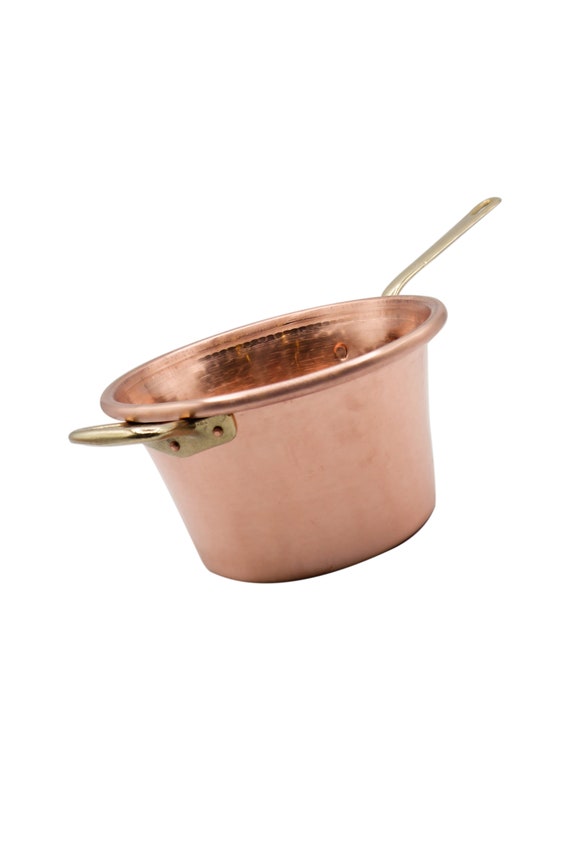This photograph features an old, small copper cooking pot set against a solid white background. The pot, tilted slightly, showcases two distinct handles: the main handle on the upper right, which is a narrow, straight stem extending outward, and a secondary handle toward the lower left, designed like a loop for a secure grip. Both handles, originally a gold or brass color, show signs of age and are attached with visible screws. The pot's exterior displays a faded copper hue, while the interior reveals a well-worn, darker brown surface, indicative of frequent use. Below the rim, there are patches of tarnish, adding to the pot's rustic charm. This simple, unembellished image captures the essence of a utilitarian kitchen tool, highlighting its aged beauty and functionality.